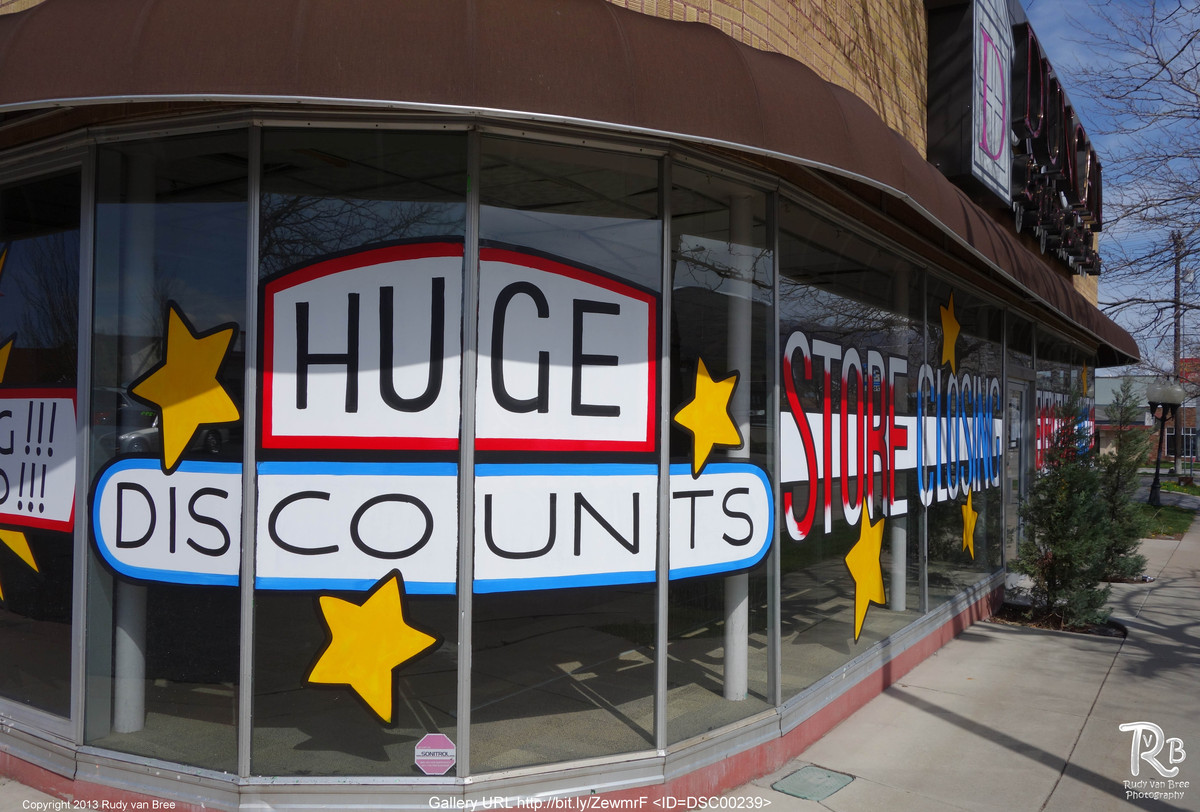This image captures the exterior of a large storefront on the corner of a two-story building, accentuated by a brown awning. The upper right-hand corner features a leafless tree reaching into a clear sky with scattered thin clouds. Dominating the scene is the storefront with expansive glass windows displaying prominent advertisements. “Huge Discounts” is written in bold black letters on a white background, highlighted with yellow stars outlined in black. The phrase “Store Closing” appears with a red-to-white gradient for "store" and blue-to-white for "closing," giving it a distinct Americana appearance. The entrance to the store features a silver door flanked by two small trees. The ground is paved with square cement tiles, and metal poles are visible through the windows. In the bottom right corner, the image is marked with the white text "Voodie Van Bree Photography," alongside an R with a V inside its loop, and a B.